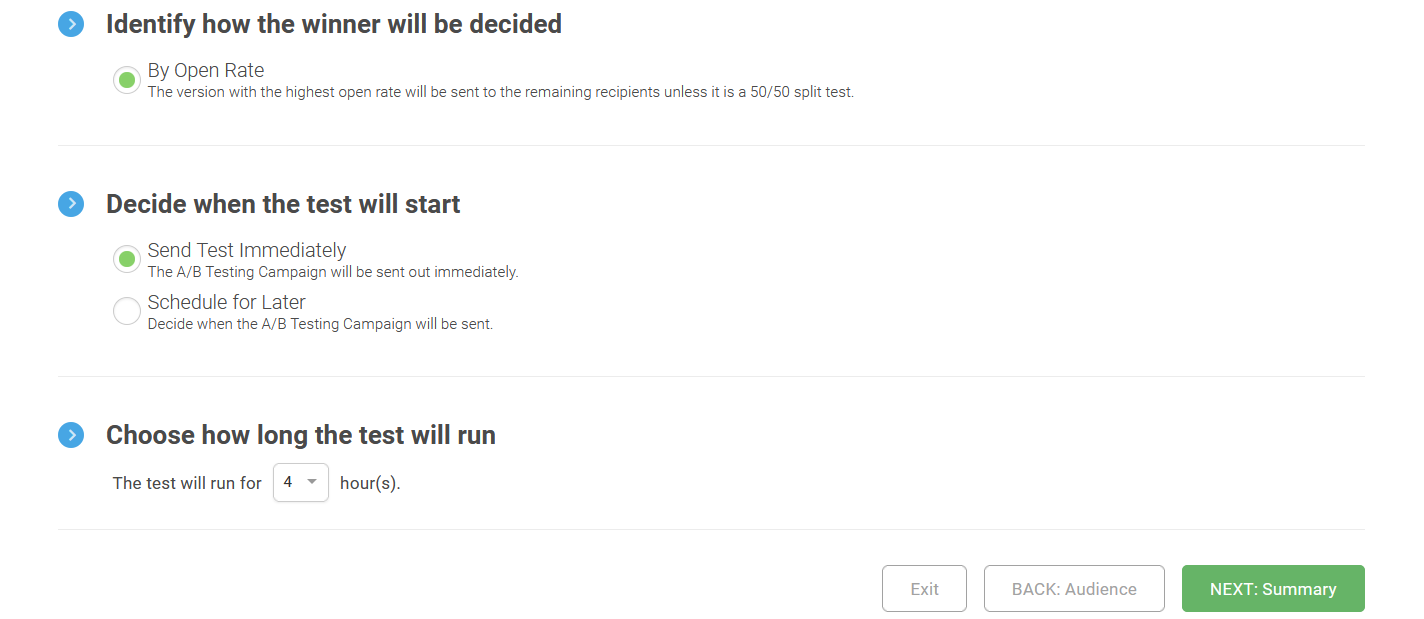In the upper left corner of the image, a bolded blue circle with a right arrow directs attention to the section titled "Identify How the Winner Will Be Decided." Below this, a green circle precedes the text "By Open Rate," indicating that the version with the highest open rate will be sent to the remaining recipients unless it is a 50-50 split test. A light gray line separates this section from the next.

The following section, also highlighted by a bolded blue circle with a right arrow, is titled "Decide When the Test Will Start." There are two options below: the first option, marked by a filled green circle, reads "Test Sent Immediately," which means the A/B testing campaign will be sent out right away. The second option, "Schedule for Later," allows the user to decide when the A/B testing campaign will be sent.

Another light gray line separates this section from the final one. The last bolded blue circle with a right arrow is labeled "Choose How Long the Test Will Run." Below this, it states, "The test will run for" followed by a drop-down menu set to "4 hours" with "hours" stylized as "hour(s)."

A thin gray line at the bottom separates the content from three navigation buttons on the bottom right. These buttons are labeled "Exit," "Back: Audience," and "Next: Summary." The "Next: Summary" button is distinguished by its green background and white font, while the other buttons are white with gray font.